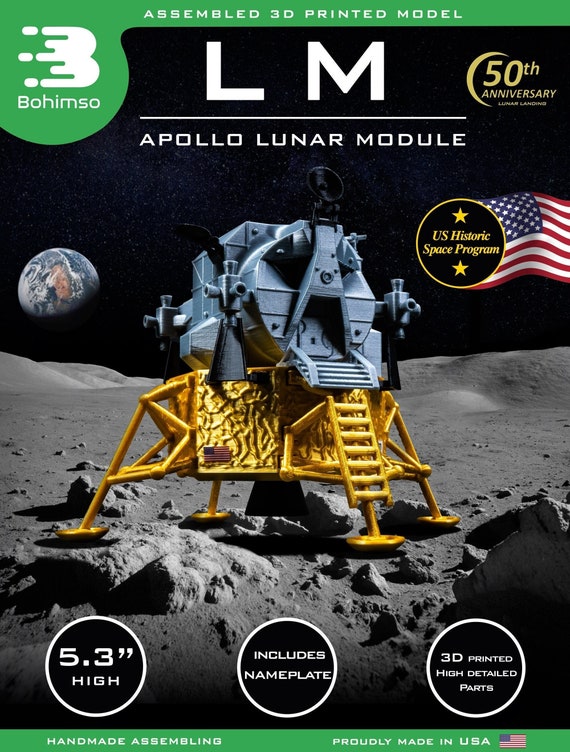The image is a highly detailed color photograph of a box containing a model of the Apollo Lunar Module. The box prominently features the text "LM Apollo Lunar Module" in bold letters at the top, and "50th Anniversary" to the right, celebrating a milestone of the U.S. Historic Space Program. The manufacturer's name, "Bohemzo," is situated to the left. The cover showcases a beautifully rendered model of the lunar module landed on the moon, featuring a distinctive golden base and a gray top with a ladder and four legs. An American flag is displayed on the module, which stands on a gray lunar surface with Earth visible against the black backdrop of space. Text on the box highlights the model's specifications, noting it stands 5.3 inches high and includes a nameplate. The model is 3D printed with high detailed parts, and it boasts handmade assembly, proudly made in the USA. There is a green ribbon at the bottom further emphasizing the craftsmanship and origin, accompanied by another American flag.